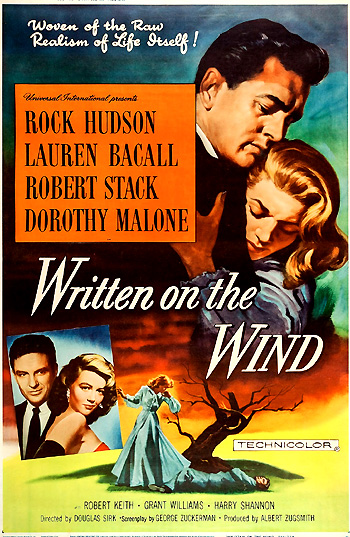This movie poster for "Written on the Wind" features vivid and dramatic imagery set against a striking color gradient background transitioning from blue to green to orange, culminating in yellow and green at the bottom. Central to the poster is the film's title, displayed prominently in white text. Above the title, the tagline "Woven of the Raw Realism of Life Itself" is showcased in cursive. 

The top left features an orange square with black text listing the film's stars: Rock Hudson, Lauren Bacall, Robert Stack, and Dorothy Malone, accompanied by the credits claiming Universal International as the presenting studio. 

Dominating the poster is an image of a handsome man with black hair in a tuxedo embracing a short-haired blonde woman dressed in a blue blouse. Positioned at the bottom left is the same couple, with the woman now attired in a red dress with long black gloves. Adjacent to this, on the bottom right, a dramatic scene unfolds with a woman standing over a fallen man by a barren tree, against an intense sunset or sunrise. 

The bottom section of the poster outlines additional credits including actors Robert Keith, Grant Williams, and Harry Shannon; and key crew members such as director Douglas Sirk, screenplay writer George Zuckerman, and producer Albert Zugsmith. The poster also highlights the film's Technicolor status, adding a note of the film's high production values.